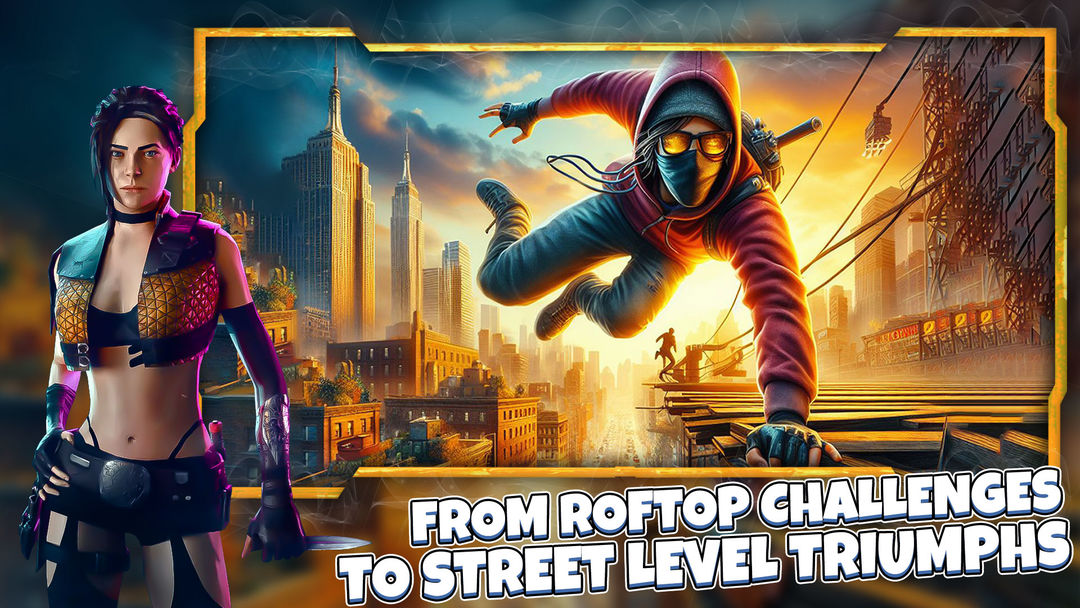The illustration is divided into two sections. On the left side, a dynamic female character stands confidently, wearing a black bikini top with a short, black and gold diamond-patterned vest. Her abs are exposed, and she has long purple and black gloves extending to her elbows. She sports a big belt, short shorts with black thong lines visible at the top, and black tights in a garter belt style. Her dark hair is parted to the left, and she wears a black necklace. This warrior-like figure has a poised yet ready-for-action stance.

On the right side, a male figure is caught mid-action, seemingly leaping across rooftops. Dressed in a red hoodie with the hood up, a white beanie, gray face mask, and black sunglasses, he exudes a sense of urgency and stealth. Gray pants and athletic shoes complete his outfit. The background features towering city buildings that evoke the atmosphere of a construction site. Below him, the text reads, "From rooftop challenges to street-level triumphs,” encapsulating a narrative of daring escapades and urban adventure. The entire scene is rendered in a vivid, animated style, hinting that it might be a promotional image or part of a larger visual story.